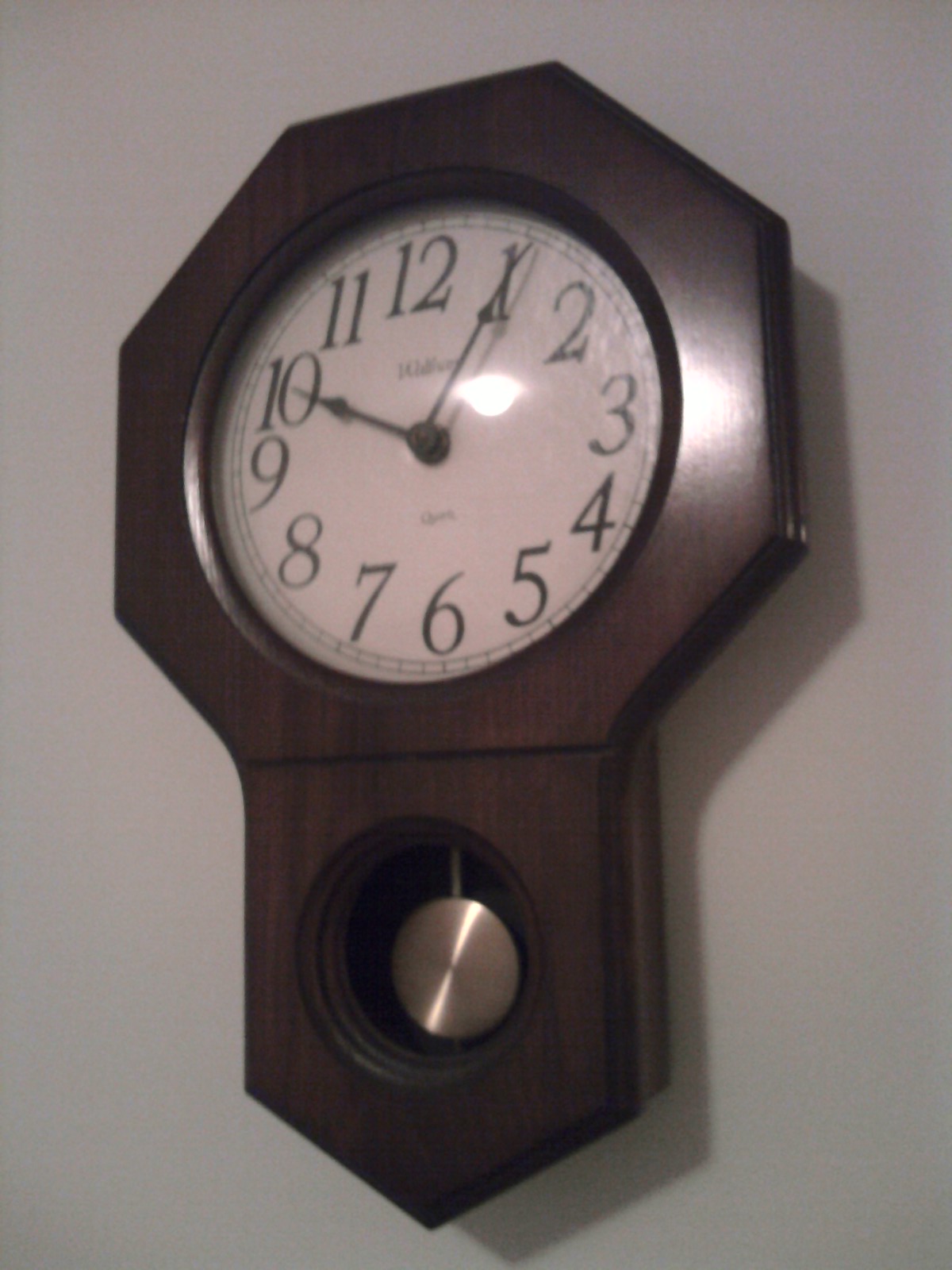A beautifully crafted wooden clock hangs elegantly on a pristine white wall, captured from a perspective slightly to the right, giving the scene a dynamic angle. The clock features a distinctive hexagonal wooden case, meticulously designed to house a prominent clock face. Below the number six, an additional angular extension of the wooden case descends, showcasing a gleaming silver pendulum that adds a touch of sophistication. The clock face itself displays large, easily readable numerals in standard English, with the time precisely set at 10:05. This image captures the timeless elegance and intricate craftsmanship of the clock against a minimalist backdrop.